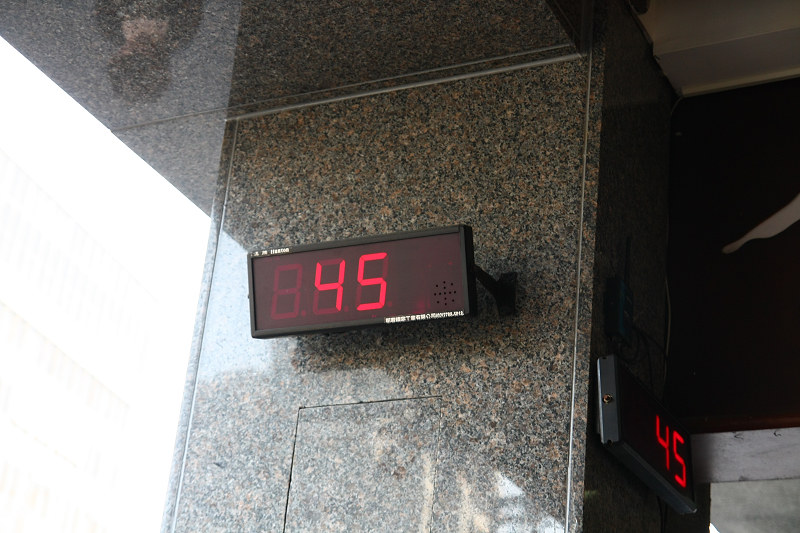The image depicts a corner within a public service building, reminiscent of a DMV. Dominating the scene is an illuminated screen displaying the number "45" in two bright spots, indicating the current number being called. The edges of the screen feature some white writing, although the exact text is unreadable. The screen is securely mounted onto a wall adorned with dark marble or granite, exuding a sense of permanence and formality. To the left, the presence of a window is inferred from the bright light spilling into the scene, creating a sharp contrast against the dimmer interior. To the right, a potential walkway suggests further pathways within the building. The viewpoint primarily focuses on the upper area, providing a direct line of sight to the numbered display and ceiling.